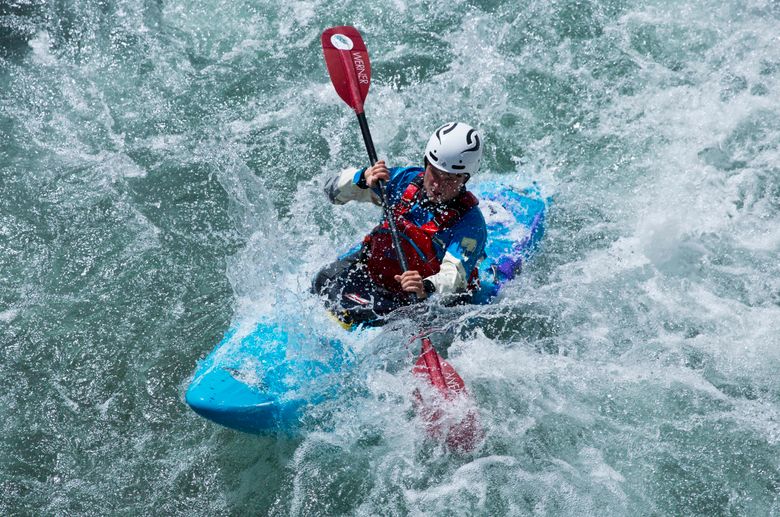A white male is intensely navigating through rough waters in a white-water rafting adventure. The turbulent waves are splashing high around him, showcasing the raw power of the river. He is in a bright blue-turquoise raft, firmly gripping red paddles as he steers through the churning rapids. His safety gear includes a white helmet with black stripes and a distinct curve pattern, a red life vest, and a blue shirt. The scene captures the thrilling challenge of the sport and is beautifully lit, indicating it was taken during the day. For more details, visit www.FEMA.gov.